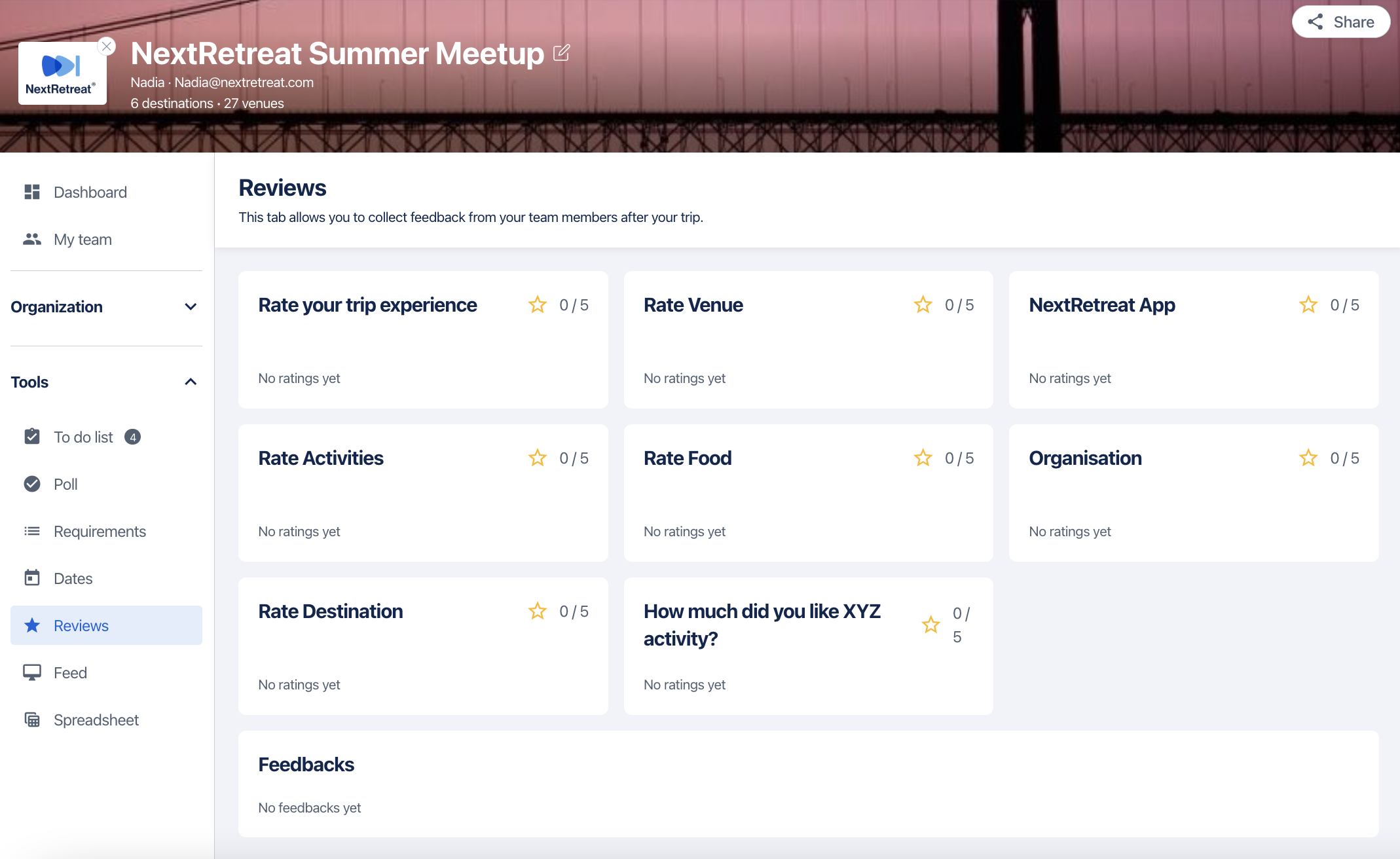The image features a screenshot of an app displayed on a MacBook, specifically an Apple laptop. The app is likely "Next Retreat," as indicated by the banner at the top of the screen which reads, "Next Retreat Summer Meetup." To the right of the banner, there is an "Edit" button. Below the banner, the meetup creator's name, Nadia, is displayed along with her contact information, "nadia@nextretreat.com." Additionally, it shows her history with six destinations and 27 venues.

The main portion of the screen is dedicated to the "Reviews" tab, designed to collect feedback from team members after their trip. The interface offers various options for rating different aspects of the trip, though currently, all categories show zero out of five ratings with no feedback yet. The categories include ratings for the trip experience, venue, Next Retreat app, activities, food, organization, and the general destination. At the bottom of the window, there is also a "Feedbacks" menu.

The layout is complemented by a sidebar on the left, though its details aren't explicitly mentioned in the voice description.